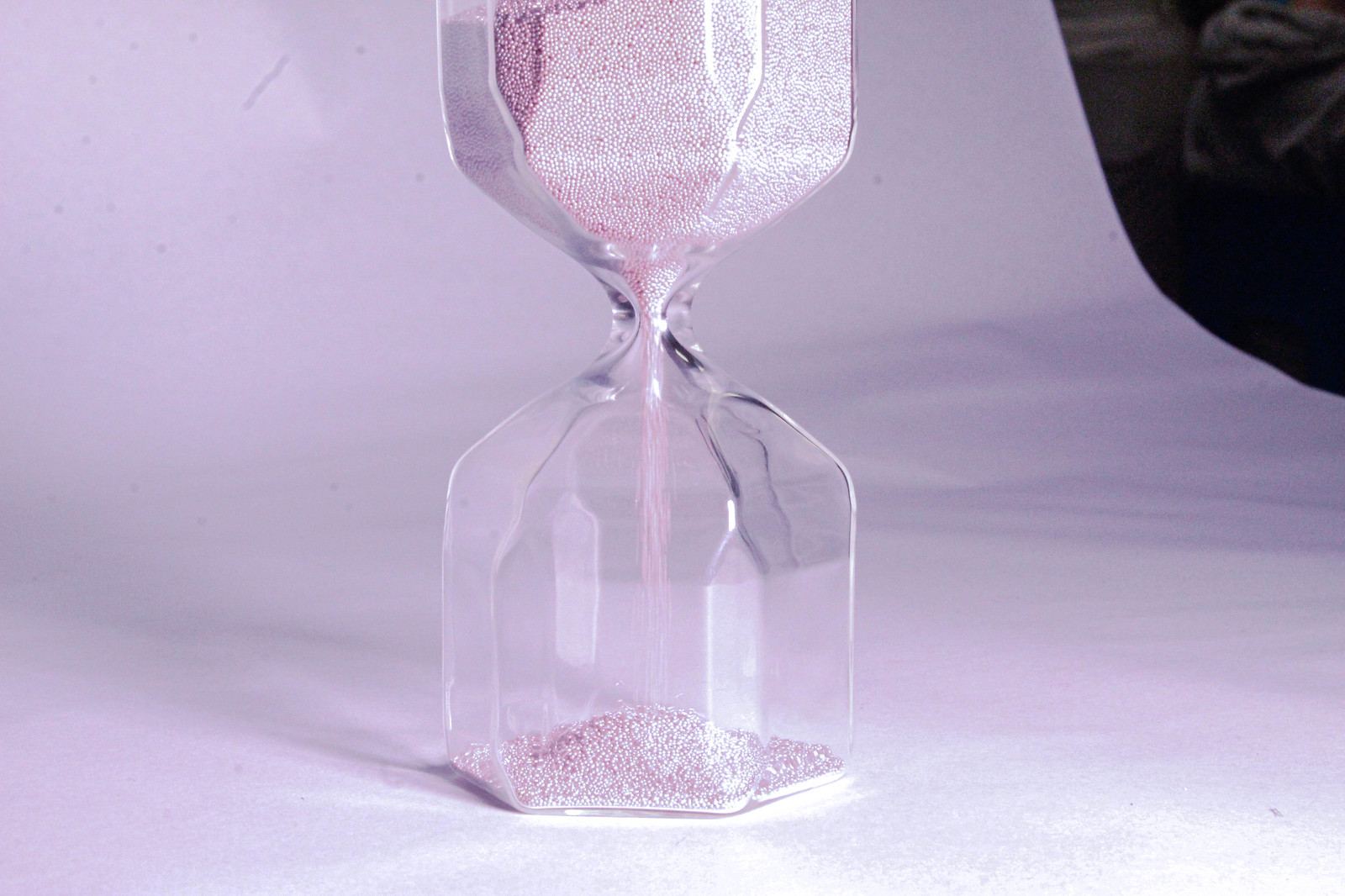The image is a captivating photograph of an unusually sculptural hourglass, which appears to be made of clear, possibly crystal, glass that reflects its surroundings. The hourglass contains pink sand, delicately trickling from the upper chamber to the lower one, with more sand in the top than the bottom, suggesting it has just begun its cycle. The backdrop is a pinkish-purple fabric that sets a dreamy, ethereal tone. Notably, there is a semicircular dark area in the upper right corner that slightly detracts from the harmonious background. The hourglass sits on a white surface that appears to blend seamlessly with the backdrop, creating a continuous, soft pink-lavender shade throughout the image. Light reflects off the right side of the hourglass, casting shadows that take on a purple hue, further enhancing the image's whimsical aura.